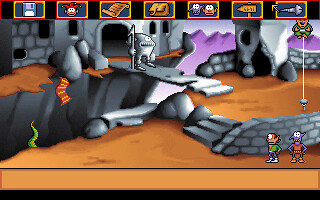This detailed screenshot from an early 90s pixelated video game features a richly textured scene predominantly in tans and grays. The setting is castle-themed with a background of purple mountains. In the lower right corner, there are two distinctive characters with big googly eyes: one is purple with orange clothing, facing the viewer, while the other, orange with brown hair and a green shirt, looks towards the castle approximately at an 11 o'clock angle. These characters stand behind a stone wall next to another bound and floating figure. Central to the scene is a stern knight-type figure, entirely gray and armed with a lance, standing guard on a narrow stone bridge that arches over a gap. This bridge connects two brown cliffs and leads to the gray castle adorned with multiple arches and doorways, overseen by noticeable stairs. At the top of the image, various game icons such as a drive, a floppy drive, a person, a joker, a document, two characters with big eyes, a sign, and a screw are visible, adding to the retro gaming atmosphere.